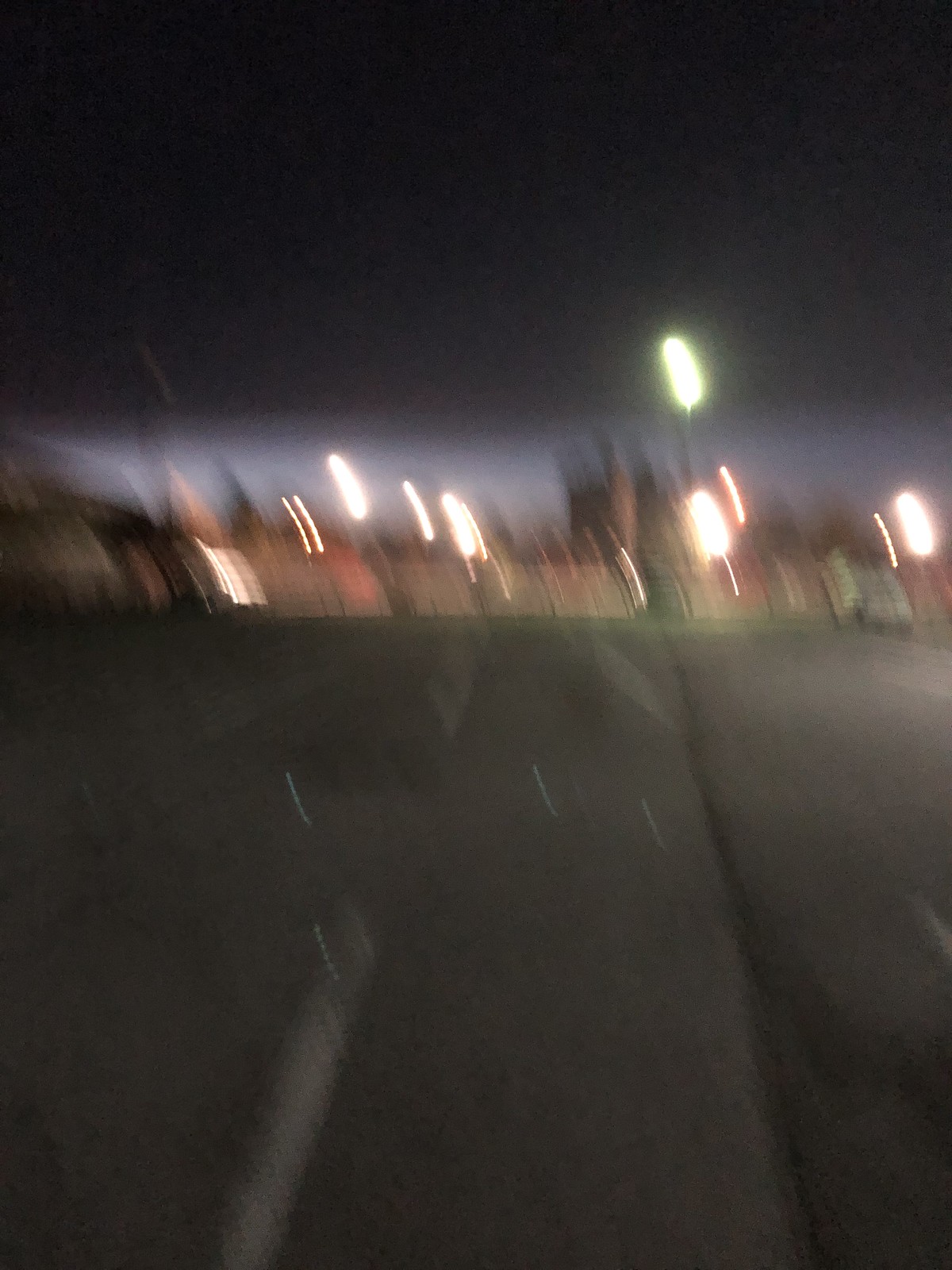This image is a very blurry photograph taken at night. The sky is completely black at the top, transitioning to a gray shade lower down. Despite the blurriness, several elongated, cylindrical lights are visible, resembling short laser beams. There are about seven of these lights; most are yellow or orange, while one, taller than the rest, is neon green. Below these lights, there's a light brown fence stretching across the middle of the image. The scene seems to be a parking lot or a street, evidenced by white lines that could be dividing spaces on a black paved surface. The area appears deserted, with a possible car faintly discernible in the left corner. Additionally, a sprawling one-story building looms in the backdrop, casting a faint illumination amidst the darkness.